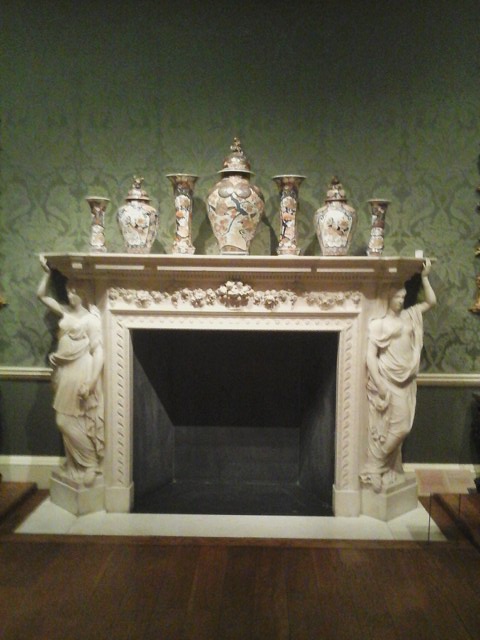This digital photograph captures an extraordinarily ornate fireplace with a highly detailed hearth and surround, possibly made of marble or a material resembling ivory. The fireplace features intricate carvings of two statues on each side, depicting women draped in loose garments similar to ancient Greek or Roman attire. Each woman has one arm raised, appearing to support the mantle above. The statues are bare-chested, with flowing shawls covering them from the midsection down. Surrounding the firebox, which is a deep, dark black square, the vertical sides and the mantle are elaborately decorated with floral carvings.

On top of the mantle, there is a sophisticated display of seven vases or urns. The central vase is the largest and most prominent, capped and richly adorned in hues of white, blue, and green. Flanking this centerpiece are two pairs of matching vases, symmetrically placed on either side, with two additional, distinct vessels occupying the outermost positions.

The background wall is adorned with intricate, grayish-cream wallpaper that features a detailed design pattern, giving an even more opulent ambiance to the setting. The wallpaper is lighter towards the base, meeting a white running board about three-quarters down the wall, above a section of grayish wood and a substantial white baseboard. The floor beneath this grand fireplace is made of dark-stained wood, completing the luxurious and historical aesthetic of the space.